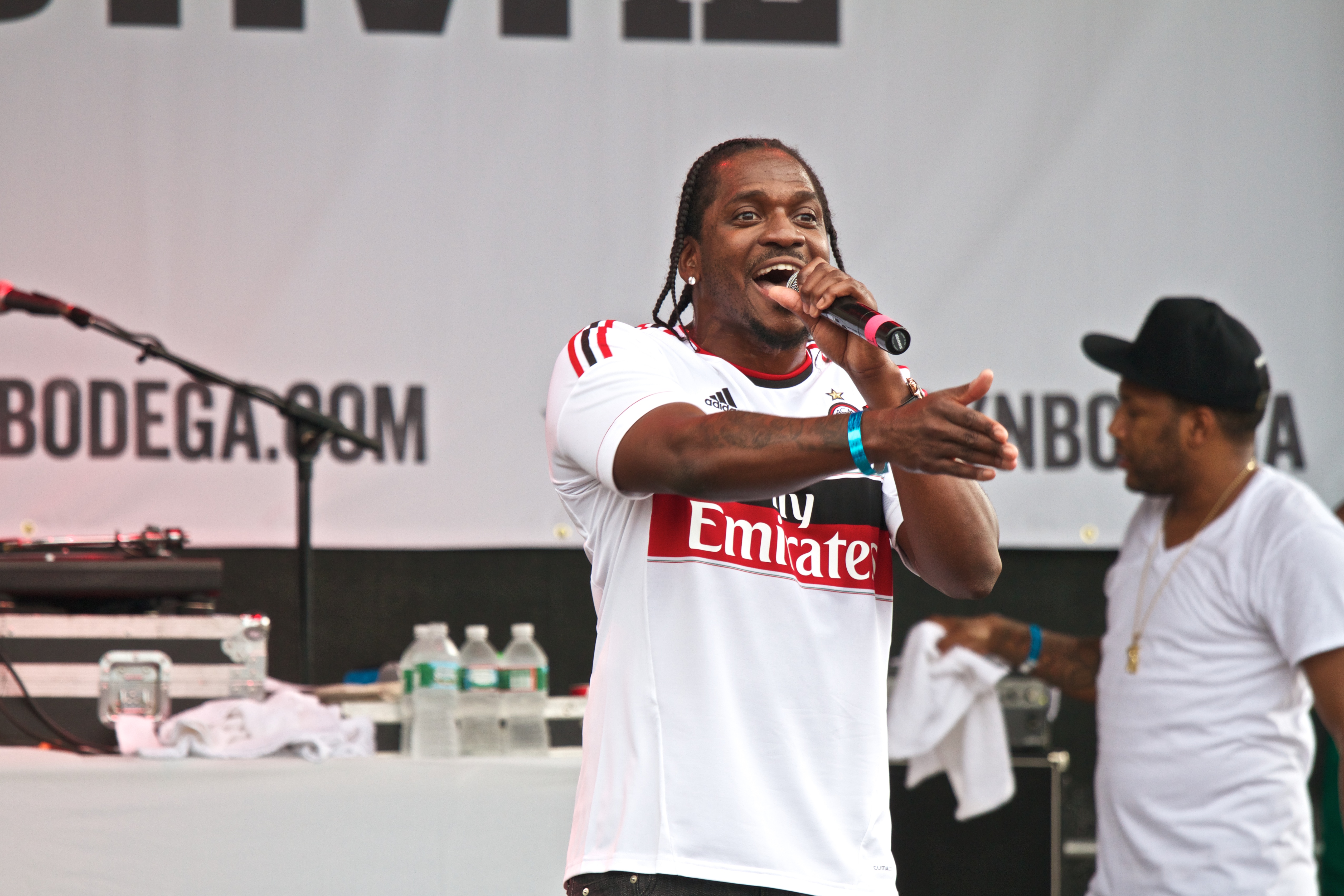The photograph captures the energetic atmosphere of an outdoor musical event. Central to the image is a black man with long black dreads and a white shirt featuring "My Emery Wright" printed in white font within a black and a red box. He stands prominently with his right arm outstretched, gesturing, while holding a microphone up to his mouth, possibly mid-performance. Behind him, to the right, another black man wearing a black cap, a white shirt, and a gold necklace holds a white washcloth. The background reveals tables adorned with white tablecloths and scattered items such as water bottles and musical equipment, indicating ongoing preparations or pauses. A partially visible white banner with black text, including "bodega.com," hints at the event's setting and sponsors. The shared elements emphasize a vibrant scene, with artists engaged in their craft amidst a supportive and organized environment.